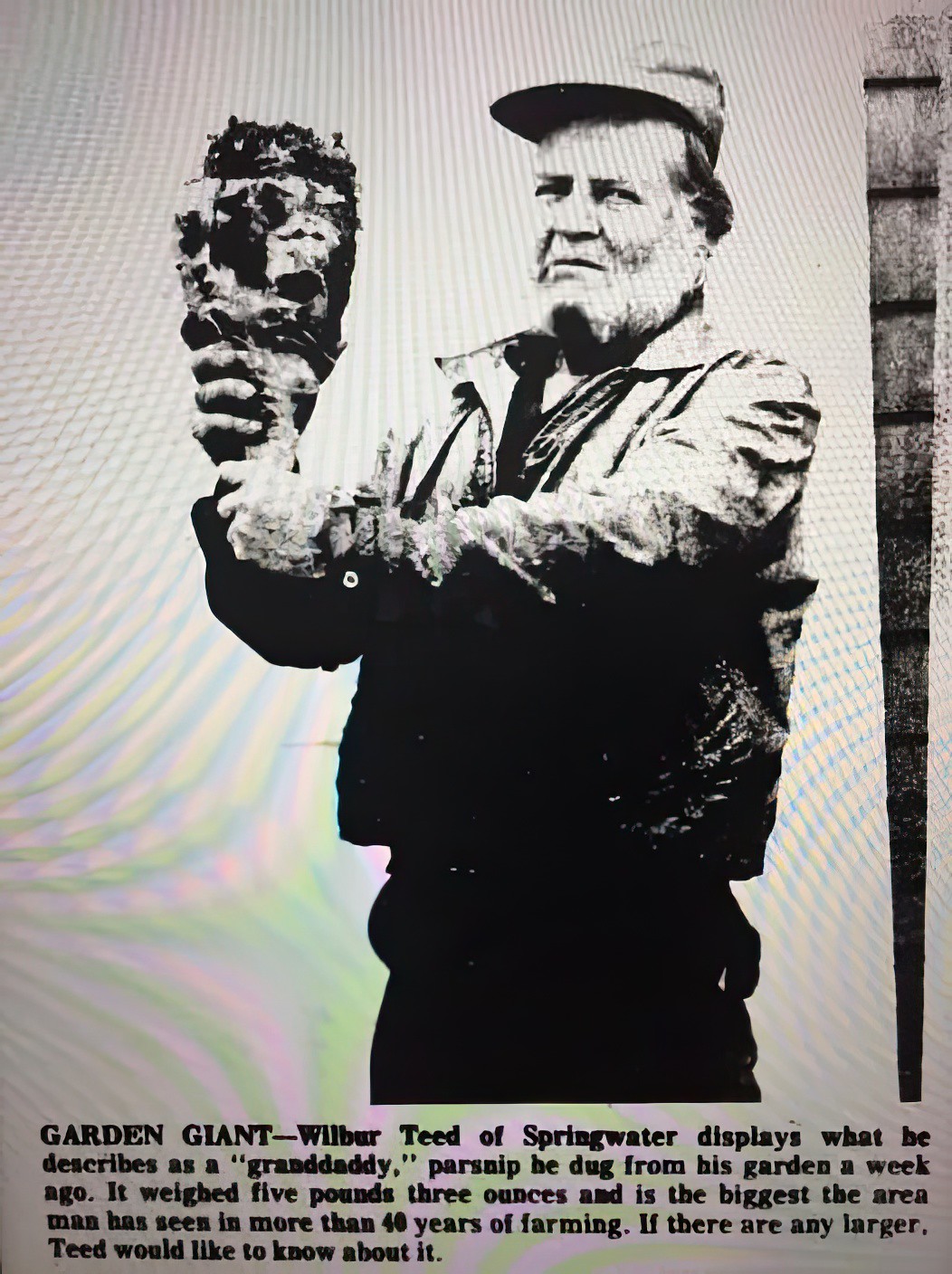In this black and white photograph, which appears to have been taken of a computer screen as suggested by some reflection, we see Wilbur Teed of Springwater prominently captured. Wilbur, a tall man with a scruffy gray beard, is portrayed in a side profile, wearing a baseball hat, a jacket, and dark pants. His hands are clutching what he describes as a "granddaddy" parsnip at chest height. The parsnip, impressive in size, weighs five pounds and three ounces, making it the largest the seasoned farmer has encountered in over 40 years of farming. The bold caption beneath the photo reads, "Garden Giant: Wilbur Teed of Springwater displays what he describes as a granddaddy parsnip he dug from his garden a week ago. If there are any larger, Teed would like to know about it."